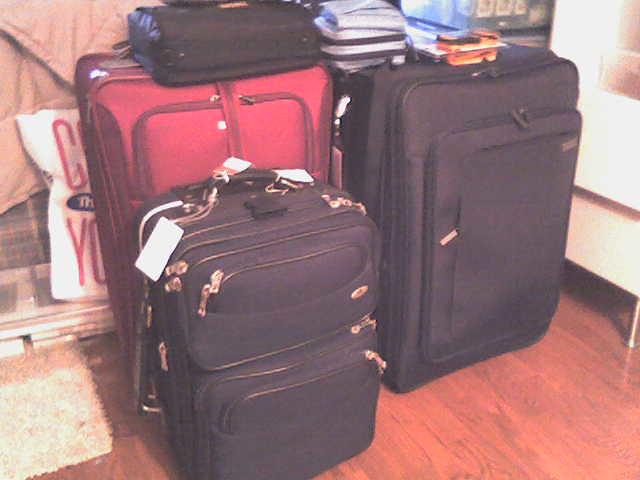This is a detailed photographic image of a room, possibly a bedroom, showcasing a collection of suitcases and travel bags. The floor is a light brown wood with a visible texture, and there is a small mat or rug in the bottom left-hand corner. The luggage is arranged centrally in the room, with three main large suitcases: a red one, a large black one, and a medium-sized black one. The red suitcase, the largest, is positioned upright with a smaller black bag laying horizontally on top of it. This smaller black bag has a gold emblem. A small black carry-on bag with gold zippers and a luggage tag is standing in front of the red suitcase. The large black suitcase next to the red one also has additional items atop it, including an orange rectangular object, possibly containing film, and some lighter-colored objects that look like a book and a piece of fabric. Behind the red suitcase is an obscured sign or pillow with partial lettering in red on a white background, displaying the letters "C" and "Y." The background also hints at a bed or couch with a light brown comforter, contributing to the coziness of the indoor setting. There are also hints of white structures to the right, which could be a window or shelving. Despite the slightly fuzzy and faded appearance of the image, either due to age or a filter, the scene clearly captures the busyness and anticipation of someone preparing for travel.